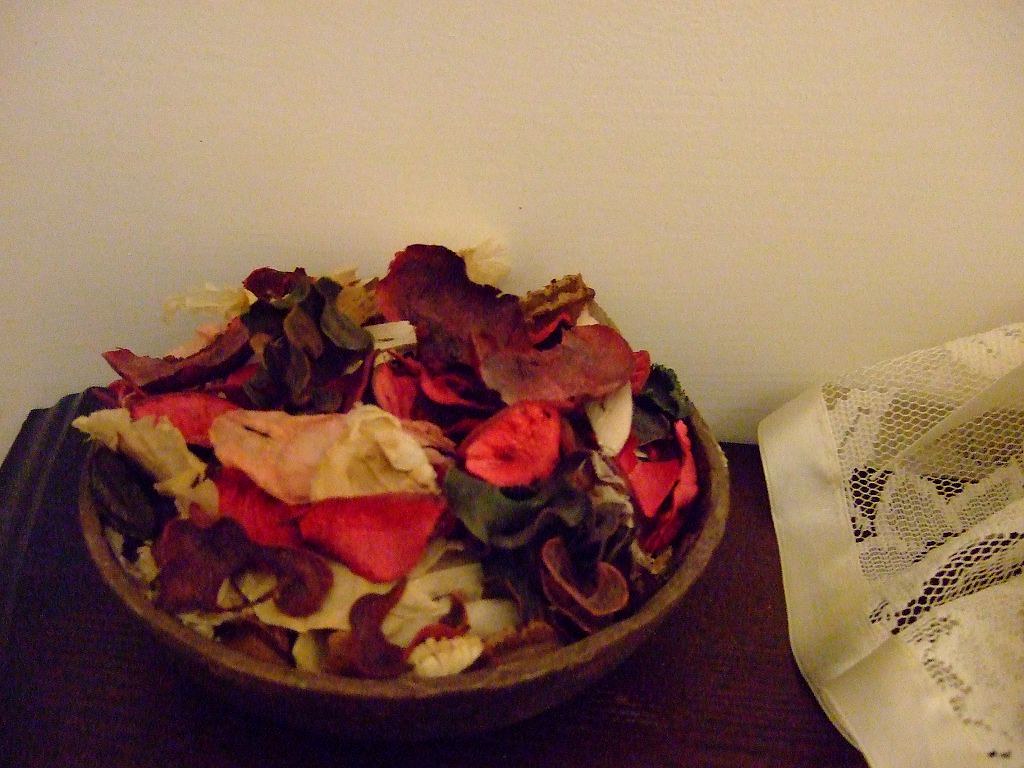In this photograph, a wooden bowl brimming with a variety of vibrant flower petals sits on the surface of a dark wooden side table. The petals, which may be intended as potpourri to enhance the room's fragrance, come in a range of colors including red from roses, white, green, purple, burgundy, tan, and brown—clearly representing multiple flower species. Behind this eye-catching array, the background features an off-white or cream-colored wall, adding to the room's serene ambiance. To the right of the bowl, a piece of fabric elegantly draped over the side table catches the viewer's attention. This fabric is a delicate mesh or doily material with intricate flower patterns and has a solid silky white hem running along its bottom edge, further enhancing the photograph’s rich texture and giving a glimpse into the room’s decor.